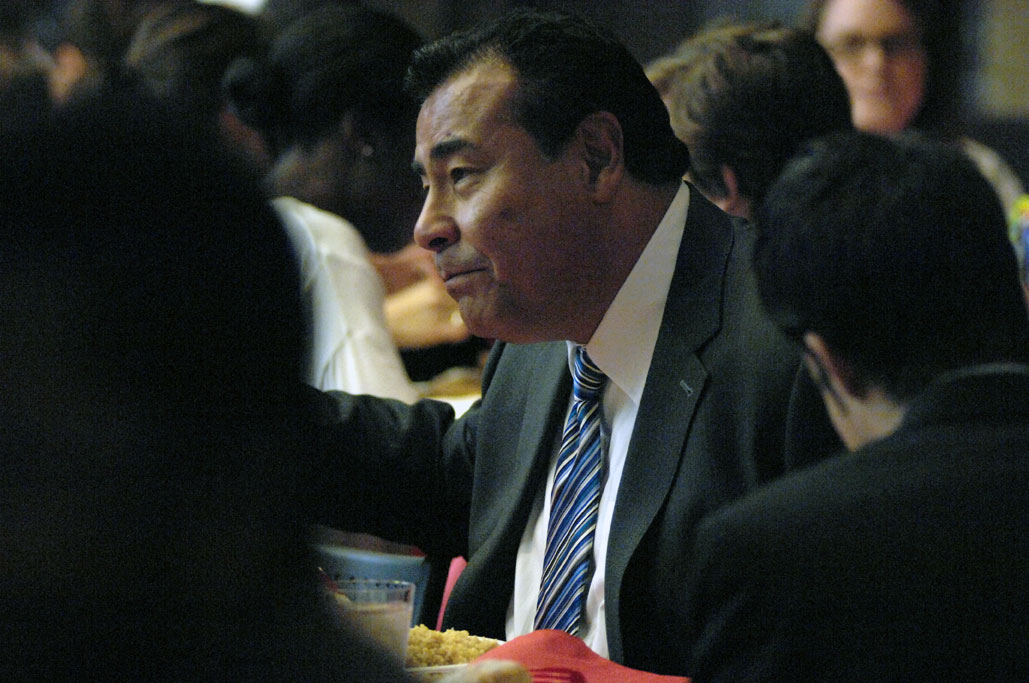The image captures a detailed scene of a gathering, likely a convention or banquet, focused on a distinguished man seated at a table. This central figure features short black hair, possibly of Asian or Samoan descent, and wears a black suit jacket over a white collared shirt, accessorized with a blue, white, and black striped abstract tie. The man appears slightly older with minor facial sagging and is depicted reaching for something on the table, partially obscured in the image. Surrounding him at the table are several other people, somewhat blurred but distinguishable. To his left is an African American woman, and in the upper right is a white woman. Another man with short black hair and a black suit jacket is visible in the background. The table itself is set with a plate of yellow food—perhaps rice or cream corn—and a red napkin. A glass of water is also prominently placed on the table, adding to the scene's banquet-like atmosphere. The overall composition and myriad details convey a bustling yet intimate social event centered around the main figure.